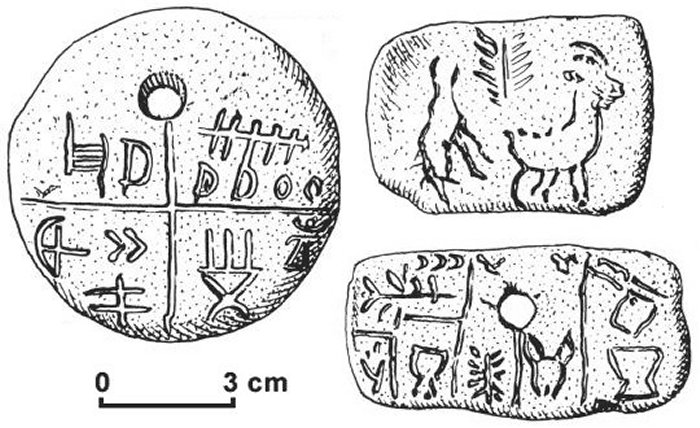This black-and-white illustration appears to be a highly detailed pen and ink drawing of three ancient artifacts, potentially from the Indus Valley civilization, made of either stone or clay. On the far left, there is a circular, flat disk about 6 centimeters in diameter, as indicated by a measurement reference below showing from 0 to 3 centimeters. The disk has a central hole near the top and is divided into four quadrants, each containing engraved symbols that resemble hieroglyphs or early writing forms. To the right of this disk are two roughly rectangular artifacts, also featuring intricate carvings. The upper rectangular object displays an engraved profile of a goat with long horns and an adjacent palm leaf-like symbol. The lower rectangular piece contains a combination of animal designs and natural motifs, including multiple engraved symbols and patterns. Both rectangular items have holes, suggesting they might have been worn as pendants. Overall, the illustration meticulously captures the texture and markings of these ancient objects, with each artifact presenting a unique set of engravings and symbols.